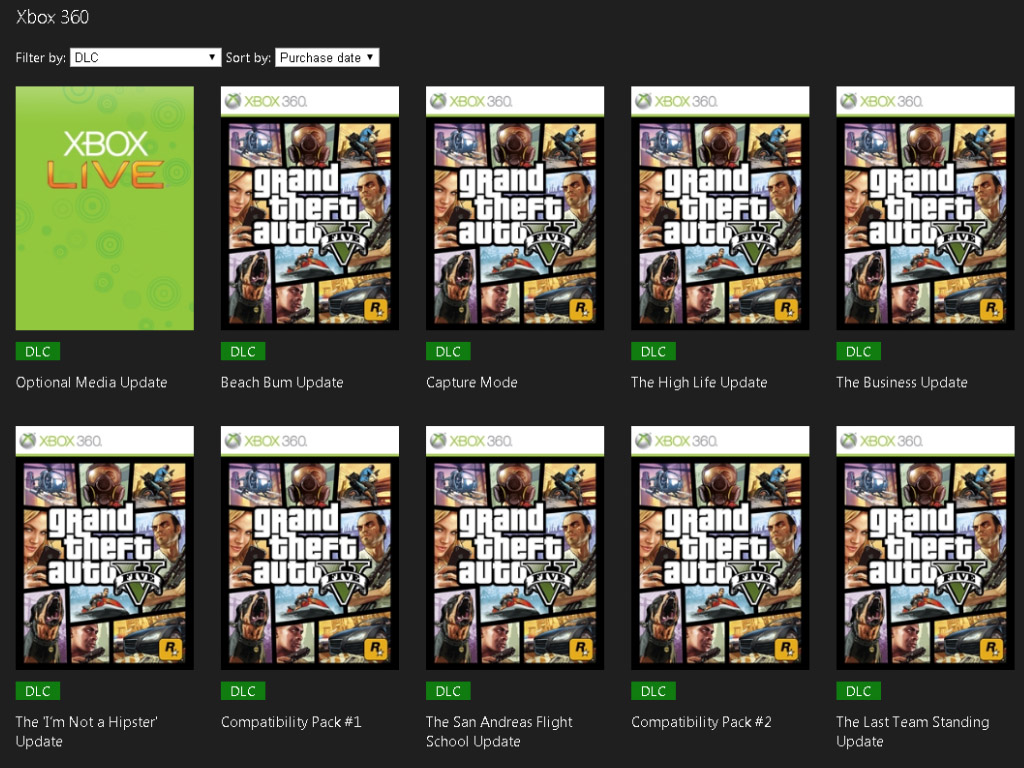The image displays an organized menu on an Xbox 360 interface, filtered to show downloadable content (DLC) sorted by purchase date. The highlighted categories include various updates such as the "Beach Bum Update," "Capture Mode," "High Life Update," "Business Update," "I’m Not a Hipster Update," and "Competitive Impact 1 & 2." Additionally, notable updates listed are the "San Andreas High School Update" and "Last Team Standing Update." The image prominently features the Xbox 360 logo and signifies Xbox Live availability. In the background, the interface showcases a dark theme with green square highlights and a selection of icons numbered from 1 to 10, most of which are related to Xbox 360 content. The scene concludes with a depiction of a helicopter and a masked figure, emphasizing the array of gaming choices available.